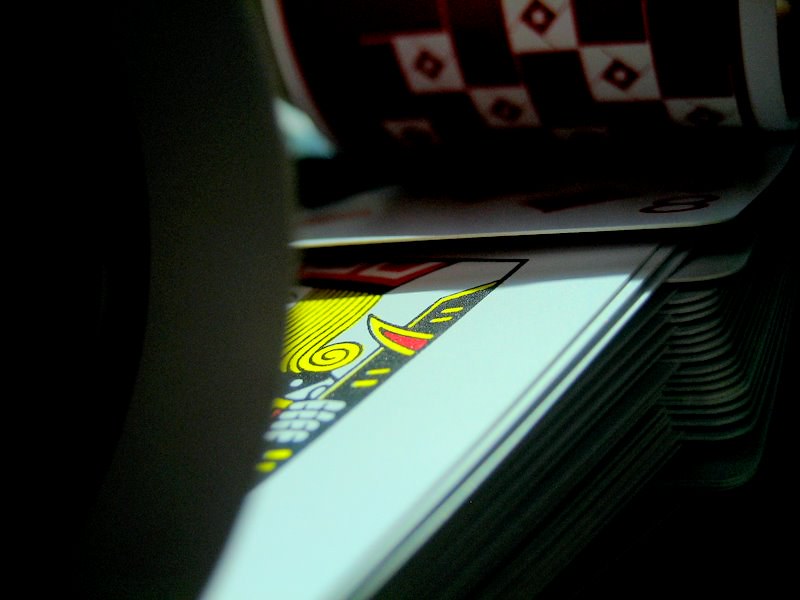The image features a close-up of two decks of cards being shuffled together on a black surface with a contrasting pitch-black background at the bottom right. The cards have a white background adorned with colored symbols and intricate artwork. The top card of the lower deck prominently displays a Joker, characterized by its yellow-blonde straight hair that curls at the side of a white face. The Joker wears a large hat decorated with red and white designs. The artwork of the Joker card is framed with a black border. 

Above the Joker card, the top card of the upper deck is revealed to be the 8 of diamonds, marked by bright red diamonds arranged around a red numeral 8. A white light casts an illumination over the bottom half of the photo, highlighting the Joker card. Meanwhile, the upper portion, including the 8 of diamonds, is shrouded in shadow. 

On the left side of the photograph, a blurry, grainy object with a gray circular border and a black interior obstructs part of the view, creating a curved outline in the frame. The entire image has a grainy texture, suggesting it may have been taken in low light or with a low-resolution camera. The two decks are mid-shuffle, with noticeable spaces between them, indicating the dynamic motion of the shuffling process.